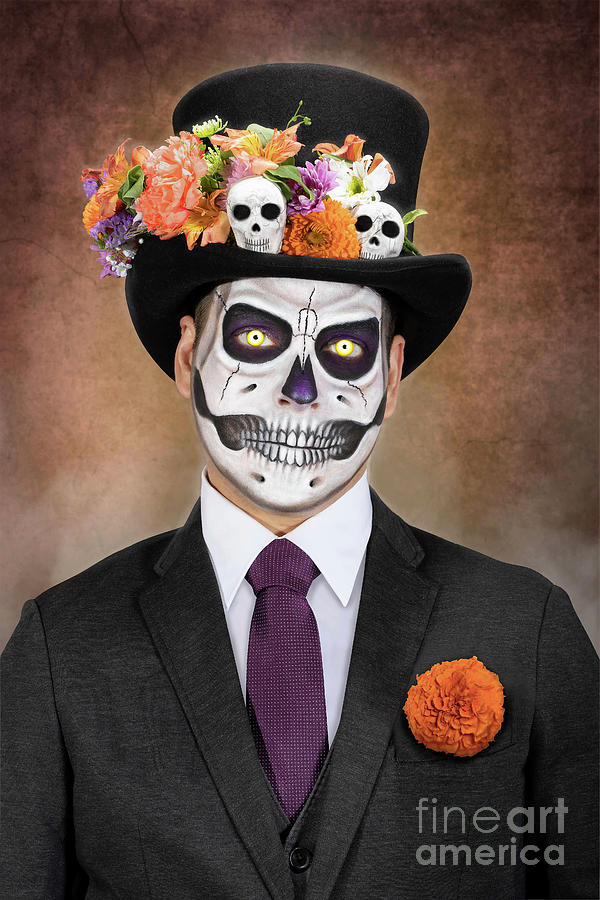In this detailed Day of the Dead portrait, the man stands out against a retro, beige-brown blotched background. His face is adorned with intricate face paint that transforms it into a white skull with teeth painted on and vivid yellow eyes, while his nose is painted a striking purple. He wears a dark charcoal suit paired with a white collared work shirt and a maroon-purple tie. An orange marigold adorns his suit pocket, adding a touch of vibrant color. Topping off his attire is a black top hat, heavily decorated with ornate flowers in shades of orange, purple, and green, along with small, silver skulls encircling the brim. The overall presentation, including the face paint, floral arrangements, and skull motifs, embodies the festive spirit of the Day of the Dead. The bottom right corner of the image features a watermark that reads "Fine Art America" in white.